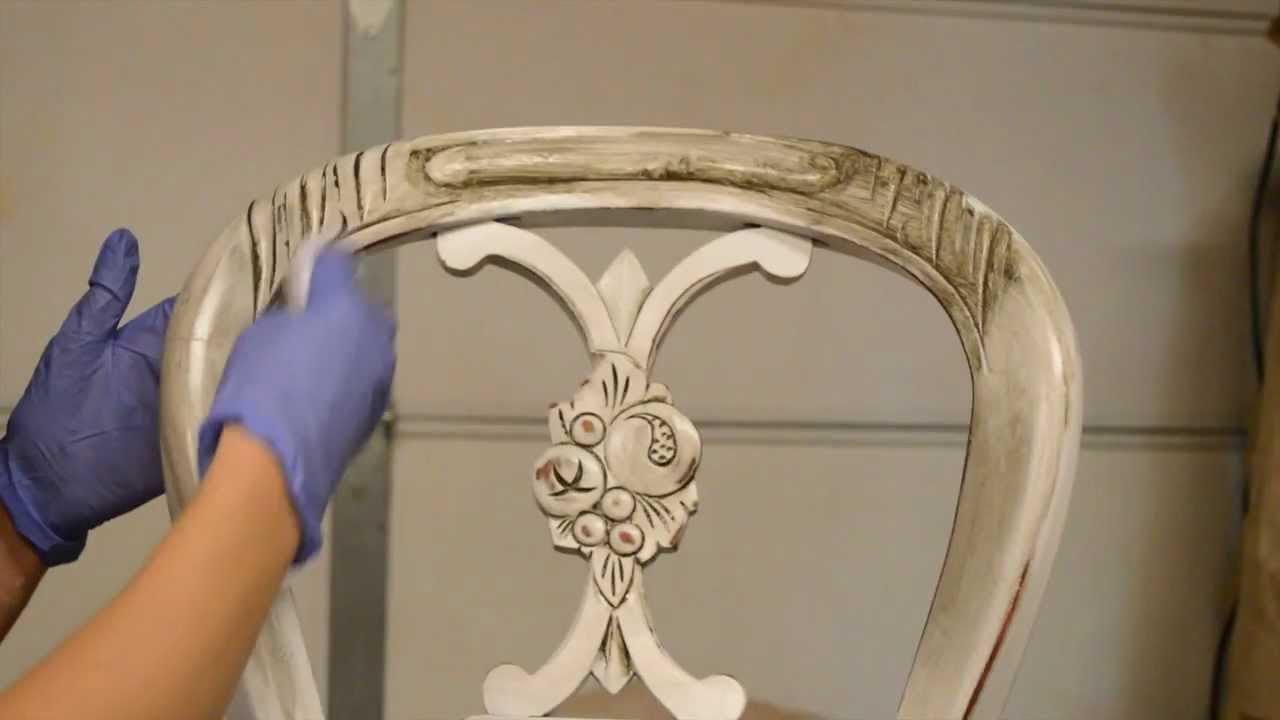The image displays the back of a pale-colored chair, seemingly antique with a unique and intricate Victorian design featuring carvings of fruits, berries, and plants. A pair of hands wearing purple gloves is seen meticulously wiping off dark varnish with a white rag, suggesting an act of cleaning or restoring the furniture. The back of the chair, supported by a pillar-like structure adorned with detailed motifs, appears slightly dirtied or marred. The background of the image consists of a wall with whitish tiles, adding a neutral backdrop to focus on the restoration work being conducted on this distinctive piece of furniture.